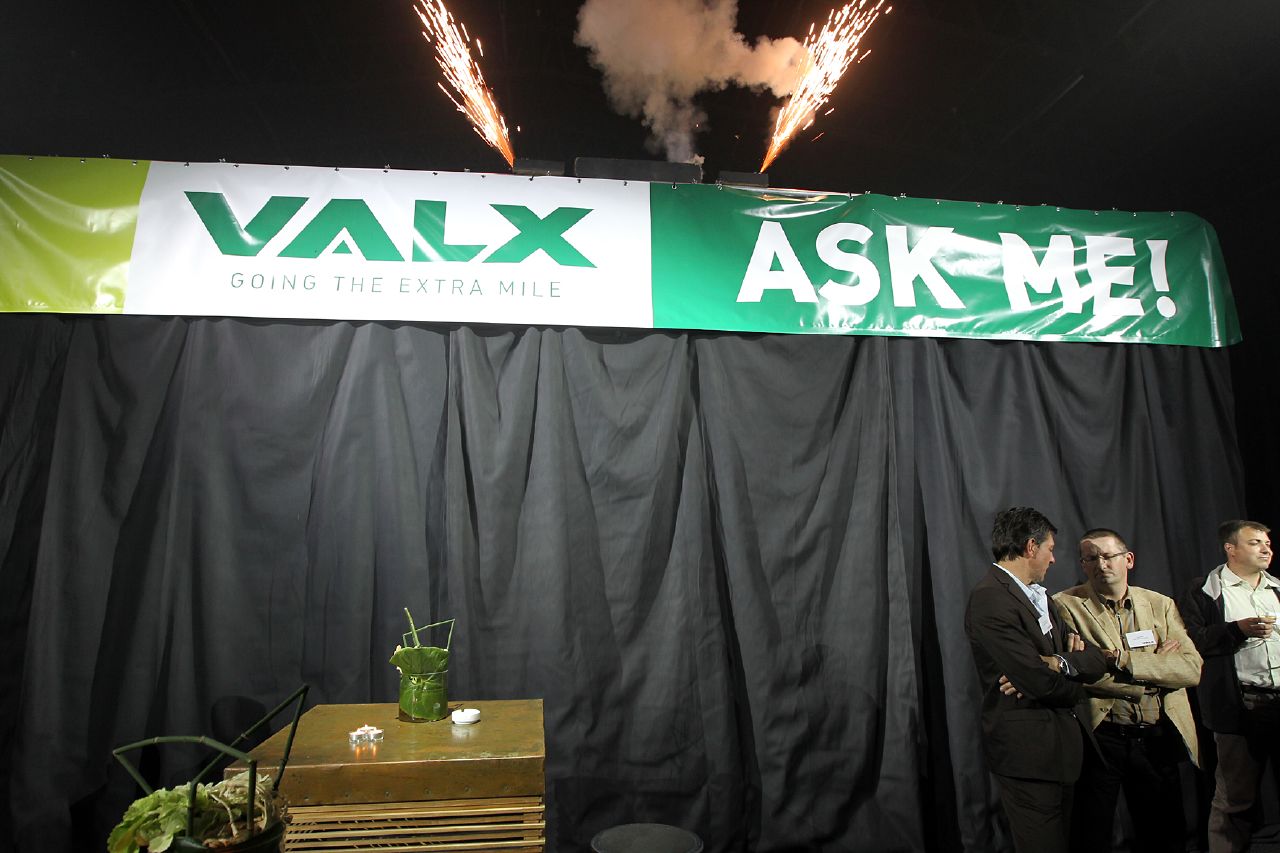The nighttime image captures a captivating scene illuminated by fireworks and a mysterious display. At the top, the dark sky is lit up by two golden fireworks, with wisps of white smoke drifting between them. A black curtain stretches from the middle of the image downward, suggesting something yet to be unveiled. Prominently displayed at the top, a green and white sign reads "VALX" in green letters, accompanied by the slogan "Going the extra mile" and an enthusiastic "Ask me!" in white. In the lower left corner, a gold-colored desk is adorned with a small green flower pot. To the lower right, three men in suit jackets and collared shirts stand together; two are engaged in conversation while the third looks to his right. This scene appears to be part of an outdoor event, likely set on a stage, with the backdrop hinting at an impending reveal behind the black curtain.